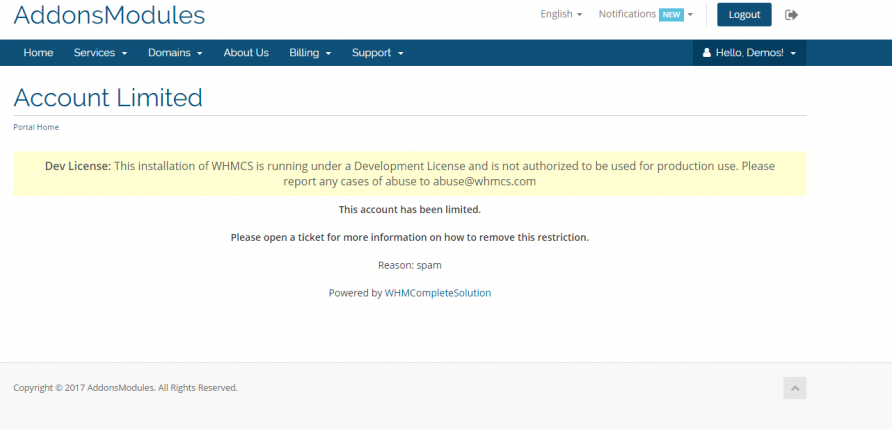The image depicts a screenshot of a website titled "Addons Modules" located at the top left corner. At the top right corner, there is a language toggle set to English, which can be changed to other languages. Nearby, there is a notification icon labeled "New" in a blue box, followed by another toggle button. A dark blue logout button with an arrow pointing to the right indicates the option to exit the account.

Below the header, a dark blue navigation bar spans the width of the page, containing links labeled "Home," "Services," "Domains," "About Us," "Billing," and "Support." On the far right of this banner, an icon of a person is displayed with the greeting "Hello, demos!" followed by a toggle button.

The main content area of the website is white, and prominently displays the text "Account Limited" in blue, followed by "Portal Home." Below this, a yellow banner states, "Dev License: This installation of WHMCS is running under a development license and is not authorized for production use. Please report any cases of abuse to abuse@WHMCS.com."

Further down, black text informs the user, "This account has been limited. Please open a ticket for more information on how to remove this restriction. Reason: Spam." At the bottom of the screen, it notes, "Powered by WHMCS Complete Solution" with a copyright notice indicating "© 2017 Addons Modules - All Rights Reserved" in the bottom left-hand corner.